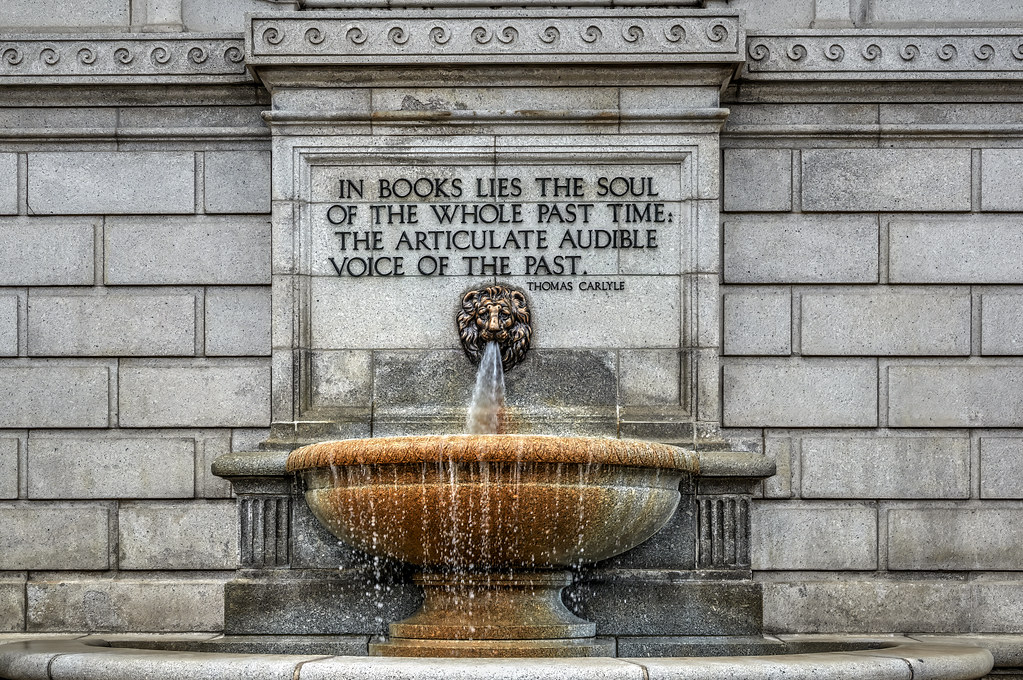The image is a landscape-oriented, color photograph of a decorated brick wall featuring a stone fountain. In the center of the wall, there is an ornate stone panel with raised lettering that displays a quote from Thomas Carlyle: "In books lies the soul of the whole past time, the articulate audible voice of the past." Just beneath this inscription is a gold-toned lion's head, from which a clear stream of water flows into a semicircular, urn-shaped bowl below. The bowl, appearing rusted and corroded, has water spilling over its edges into a larger container beneath. The overall scene has a detailed, representational realism, capturing the texture and aging of the materials as well as the flowing movement of the water.